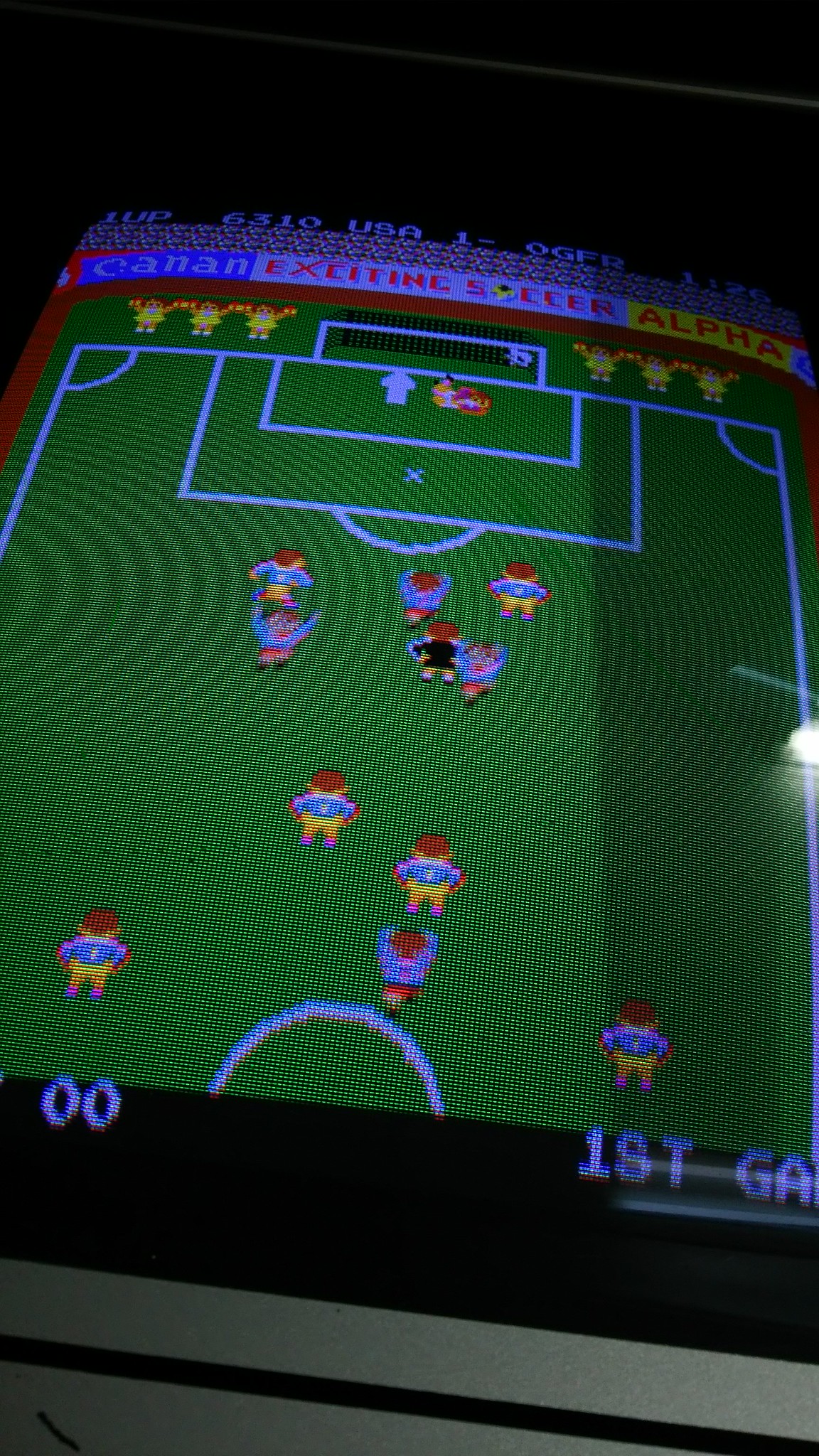In the image, we are viewing the screen of either a phone or a laptop, displaying a video game with notably low resolution. The game appears to depict a soccer match. At the bottom of the screen, blue text indicates the score as "0 - 0" for the first half, referred to as "GA," likely meaning "game." The players are seen on what seems to be a soccer field, though no soccer ball is visible in play. We can see the backs of several players, all donned in blue tops with yellow and orange shorts, running towards what looks to be the goal area. The field has a green surface. A referee, distinguishable by their black top, is also visible on the field. At the top of the screen, the title "Exciting Soccer" is displayed. The teams are identified as "Canaan" on the left and "Alpha" on the right. Additionally, six cheerleaders dressed in yellow outfits are facing the audience, adding to the lively atmosphere of the scene.